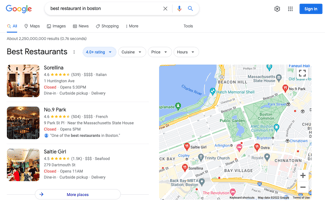This image captures a close-up of a Google search results page, albeit out of focus and blurry. At the top left corner, the iconic Google logo is prominently displayed. Dominating the center of the page is the search bar, containing the partially readable query "best restaurant in..." with the rest obscured, possibly indicating "Boston" based on context clues. To the upper right, the "Sign in" button is clearly visible.

Just below the search bar, a row of category tabs is stretched horizontally, including "All," "Maps," "Images," and other categories that are not fully discernible due to the image's lack of clarity. The main content section features a list of the top three restaurants corresponding to the search query. Each entry includes a thumbnail image, the restaurant's name, its star rating, current closed status, and details on when it will next open.

On the far right side of the page, there's a small, heavily pixelated map dotted with location pins indicating where these restaurants are situated. Unfortunately, the poor image quality compromises readability and makes it challenging to ascertain specific details from both the map and the listings. This snapshot is a Google search result page focusing on restaurants, captured in a blurry and unfocused state, complicating the full comprehension of the information presented.